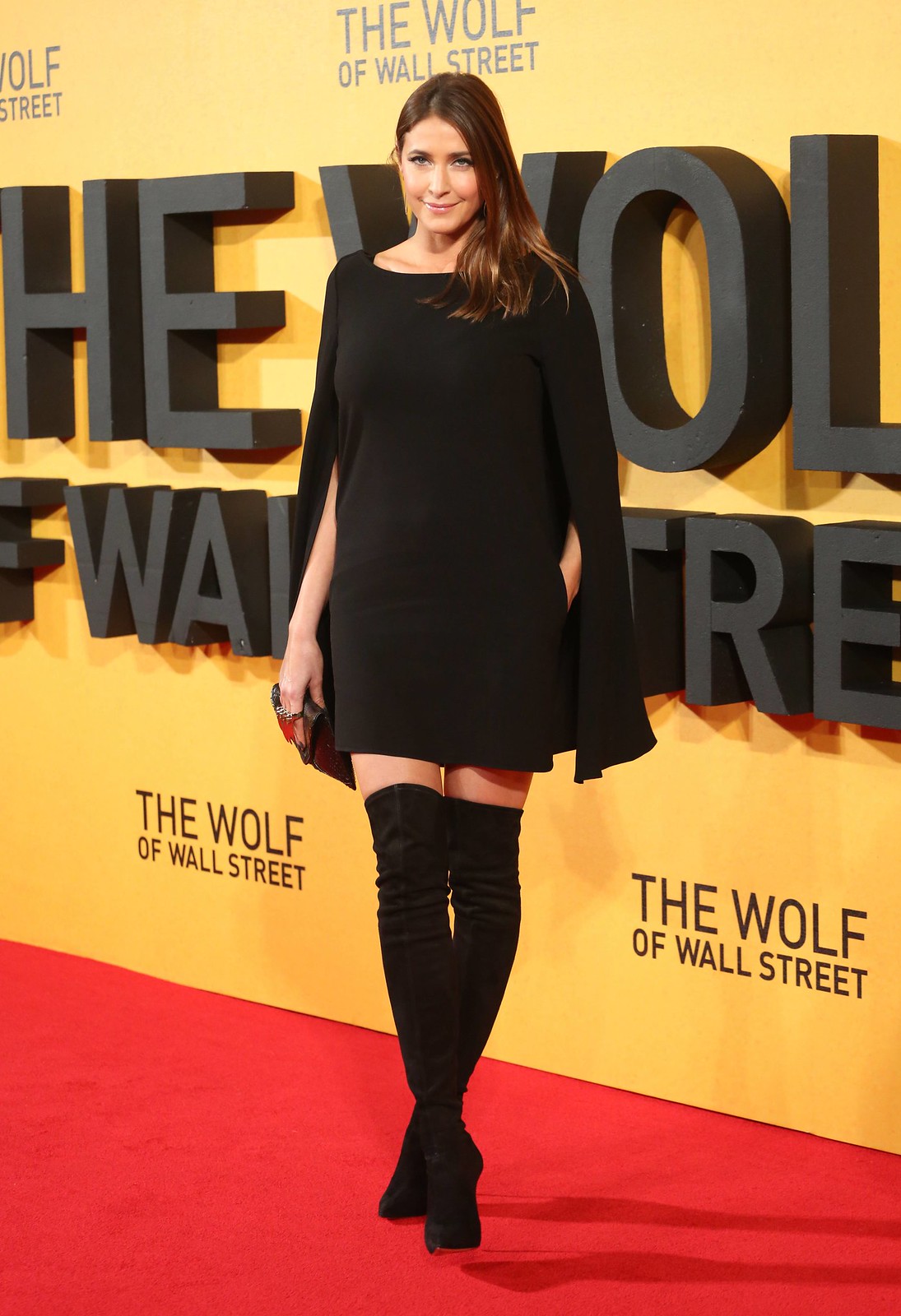In this red carpet photograph, a beautiful young woman, possibly attending a premiere, stands confidently in front of a large yellow backdrop adorned with the title "The Wolf of Wall Street" in both very large 3D letters and smaller, repeated print. Though the full title in 3D is partially cropped out, the smaller print in black, capitalized letters is clearly visible on the pale gold background. The woman has medium to light brown hair that flows around her shoulders and down her back, complementing her light makeup and closed-mouth smile. She is wearing a striking black mini-dress that features open sleeves, giving it a cape-like appearance, and thigh-high black boots made of a soft material, which highlight her slender legs. Accessorizing with rings on her right hand, she holds a small black clutch purse, with her other hand tucked casually into a pocket. She stands poised and elegant on the red carpet, encapsulating the glamour and excitement of the event.